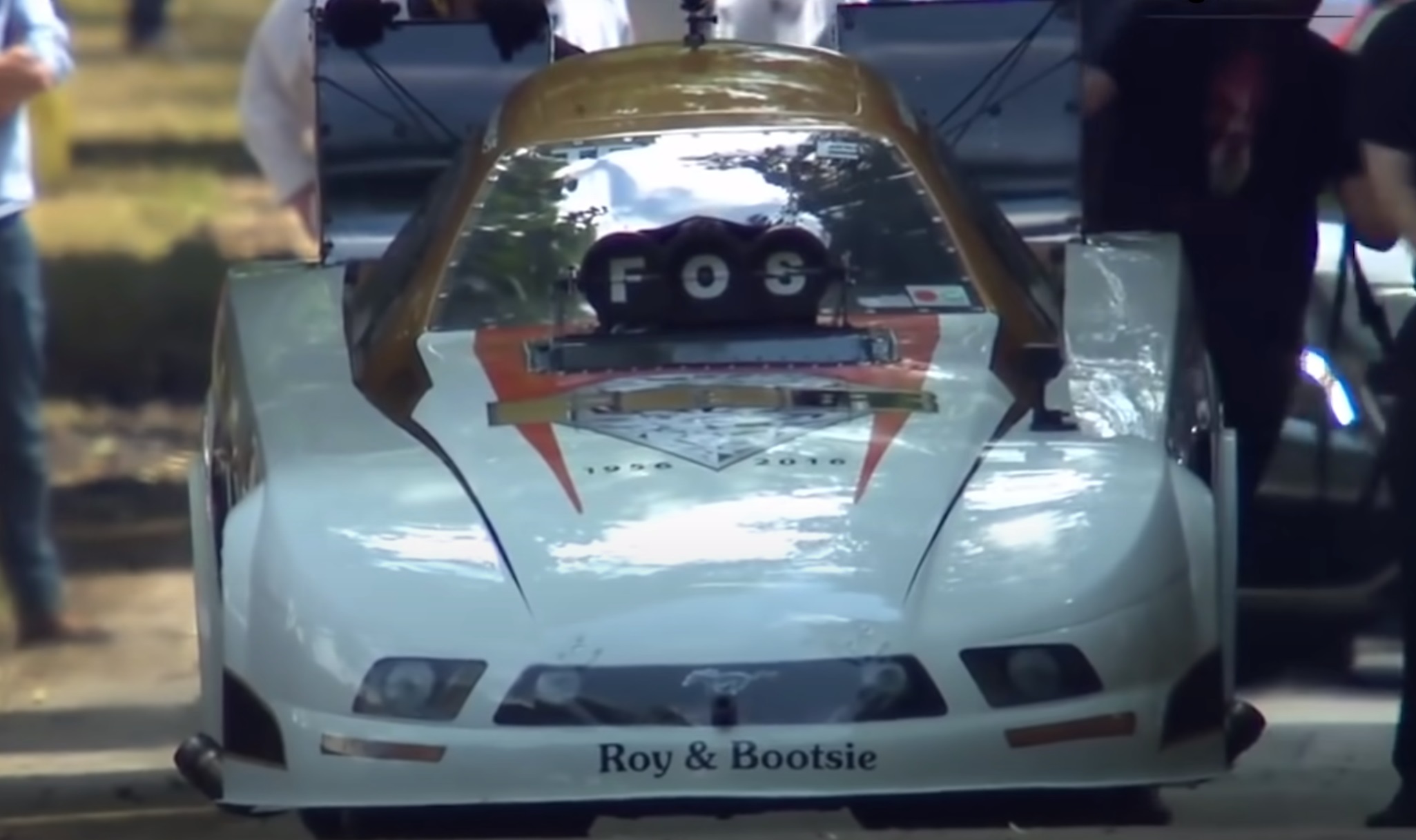This photograph captures the front view of a sleek, narrow race car, resembling a Mustang, prominently displayed against a backdrop of grass and onlookers. The car is predominantly white with a distinctive golden-brown, highly reflective glass canopy forming its roof. The word "FOS" is emblazoned across the center of the hood in white letters on a black background, possibly surrounded by other painted promotional elements that are less discernible. Below, at the very base of the vehicle's front end, the names "Roy and Bootsy" are clearly visible. The vehicle's design includes flailing elements and pipes emerging from the front hood, likely part of its exhaust system. Surrounding the car, the lower halves and limbs of several observers can be seen, indicating the car is attracting attention. The compact, single-seat design suggests it is a specialized speed racer, equipped with components like flaps and a parachute for braking at high speeds. The tires and wheels are fully encased by the car's plastic shell, enhancing its aerodynamic profile.